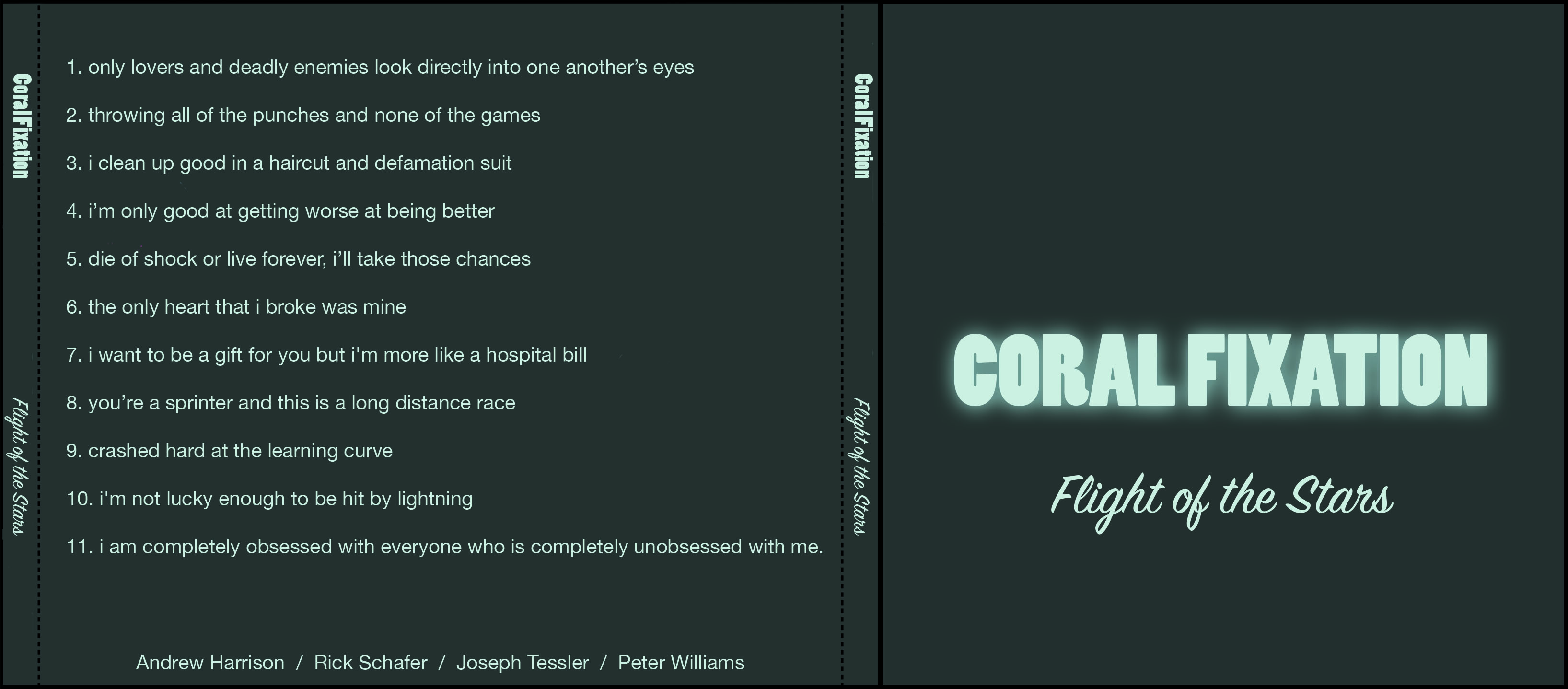The image portrays an opened book with both covers visible. The book has a grayish-brown cover accented by light greenish writing. Dominating the right cover, “CORAL FIXATION” is boldly inscribed in all caps, blocky letters. Below this title, the subheading “Flight of the Stars” is elegantly penned in a script font. 

On the left side, there's a list numbered from 1 to 11, written in a clean, sans-serif font. Here are the entries:
1. "Only lovers and deadly enemies look directly into one another's eyes."
2. "Throwing all of the punches and none of the games."
3. "I clean up good in a haircut and defamation suit."
4. "I'm only good at getting worse at being better."
5. "Die of shock or live forever, I'll take those chances."
6. "The only heart that I broke was mine."
7. "I want to be a gift for you, but I'm more like a hospital bill."
8. "You're a sprinter, and this is a long-distance race."
9. "Crashed hard at the learning curve."
10. "I'm not lucky enough to be hit by lightning."
11. "I am completely obsessed with everyone who is completely unobsessed with me."

Additionally, the phrase “Coral Fixation Flight of the Stars” appears in a much smaller font, both in the middle and along the left side column, oriented sideways. At the bottom, the names “Andrew Harrison / Rick Schaefer / Joseph Tesler / Peter Williams” are listed, suggesting possibly authors or contributors. The entire text on the left side is in lowercase, white font against the gray background.